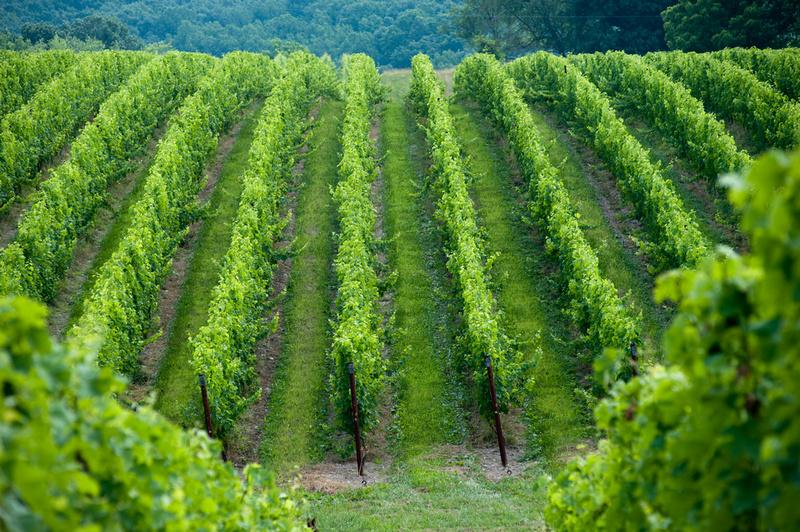The image is a landscape color photograph capturing a meticulously organized farm field on a hillside. The primary elements of the scene are the rows of vibrant green crops, likely grapevines, each supported by black wooden posts. These rows extend horizontally from left to right and are separated by grassy paths, creating a structured and verdant pattern. The crops are planted on a gently sloping terrain, which descends from the top of the image towards the viewer at the bottom, giving an impression of depth. In the foreground, each row is marked by a prominent brown or black wooden post. The hillside planting allows the rows to gradually disappear at the ridge toward the top of the image. The background features additional green vegetation and trees, their blue-green hues adding to the natural ambiance. The photograph reflects a realistic, representational style, emphasizing the detailed and orderly nature of the cultivated landscape.